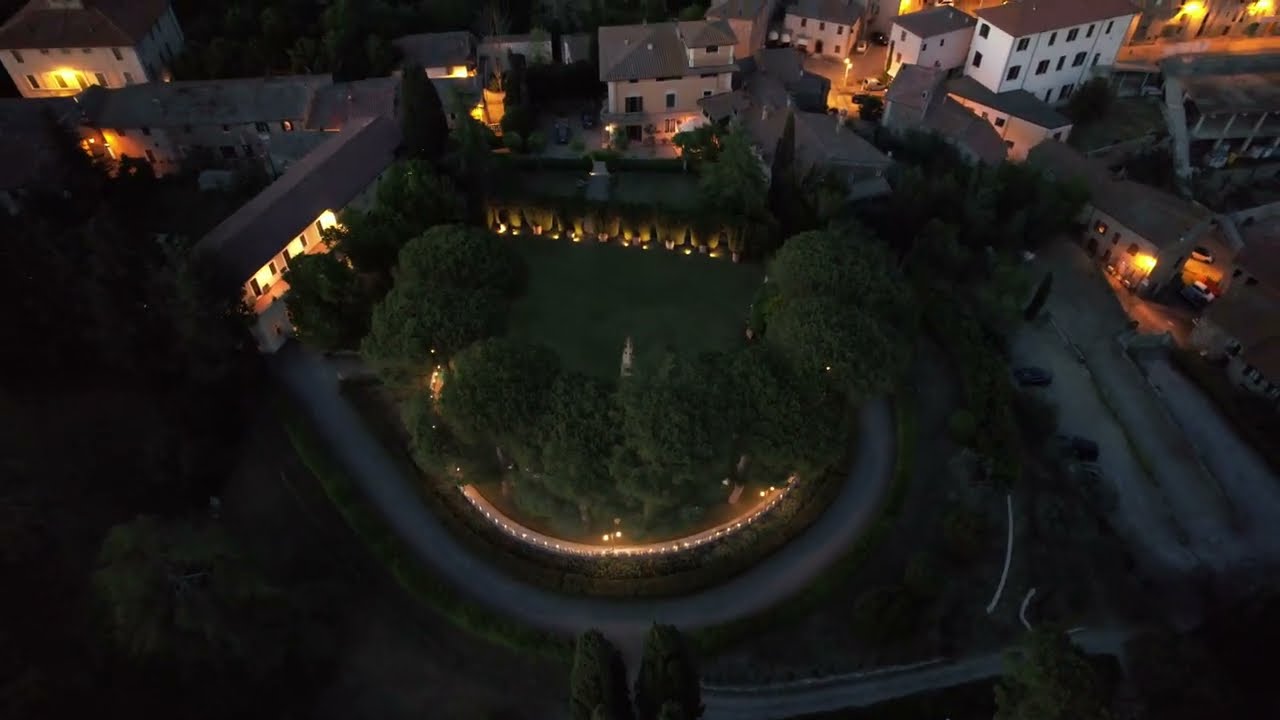The image is a clear, nighttime aerial photograph of a neighborhood, possibly taken from a drone or helicopter. At the heart of the image lies a semicircular park, bordered by large trees along its arch and interspersed with green grass. Illuminated pathways highlight the edges of the park, and towards the back, a wall with upward-pointing lights can be discerned. The scene is bathed in various hues, including green, beige, brown, red, and white, adding to its vibrant nighttime appeal. Surrounding the park, a residential area composed of numerous white and beige Mediterranean-style houses extends into the background and flanks both sides. The homes emit a warm glow that complements the well-lit streets and pathways. On the right side of the image, a gravel car park is visible with several cars parked diagonally. Overall, this detailed and well-lit image offers a comprehensive view of a quaint and organized neighborhood centered around a charming, tree-lined park.